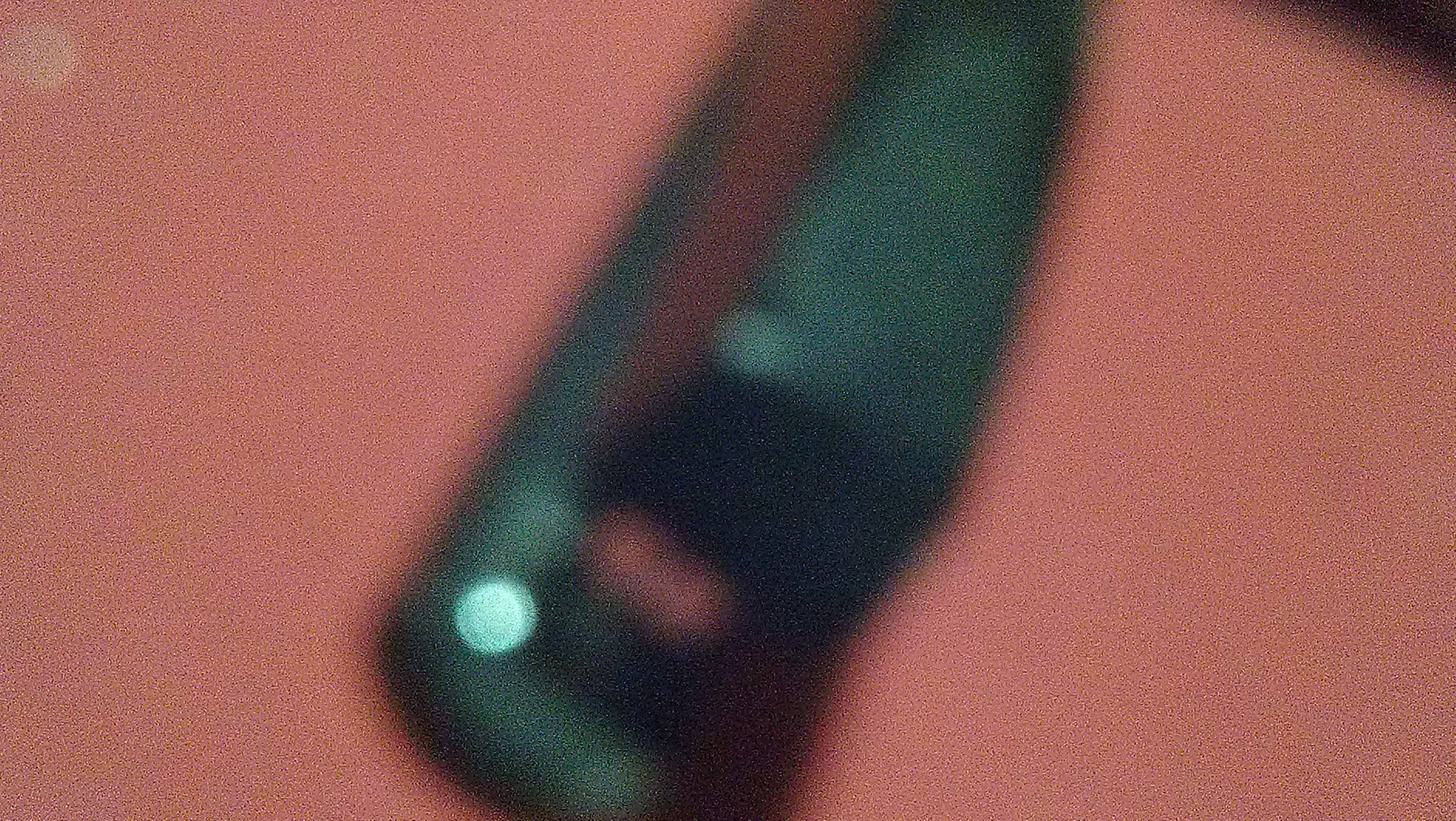The image, though extremely grainy and blurry, depicts what appears to be a stapler. Upon closer examination, you can make out the distinct features of a stapler, including its black base and the separable parts that open up for stapling. The identifying element is the prong at the front where staples are dispensed. The stapler seems to rest on a surface with a pinky mauve color, which could be a desk or dresser. In the image's top right corner, there's a black section, and another corner features a noticeable orb. Additionally, another orb reflection is visible on the stapler's base, which may be the part used for spreading out staples.